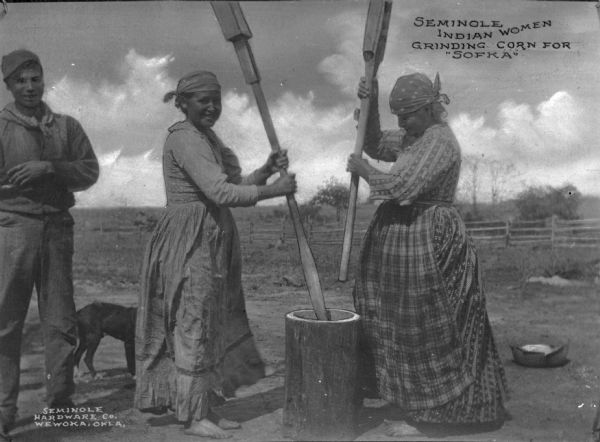This detailed black-and-white photograph, likely from the early 1900s, captures a scene titled "Seminole Indian Women Grinding Corn for Sofka" as written at the top. The image shows two women diligently engaged in grinding corn using large wooden mallets, working over a hollowed-out log, presumably to prepare Sofka, a traditional dish. Both women have their hair tied back with bandanas and are dressed in long-sleeved shirts, skirts, and aprons. To the left, a man stands with a relaxed posture, smiling at the camera, while a dog is partially visible behind him. The background features a gray, likely cloud-streaked sky, a wooden fence, sparse desert-like vegetation, and scattered trees and tumbleweeds, providing a rustic backdrop to this historical snapshot.